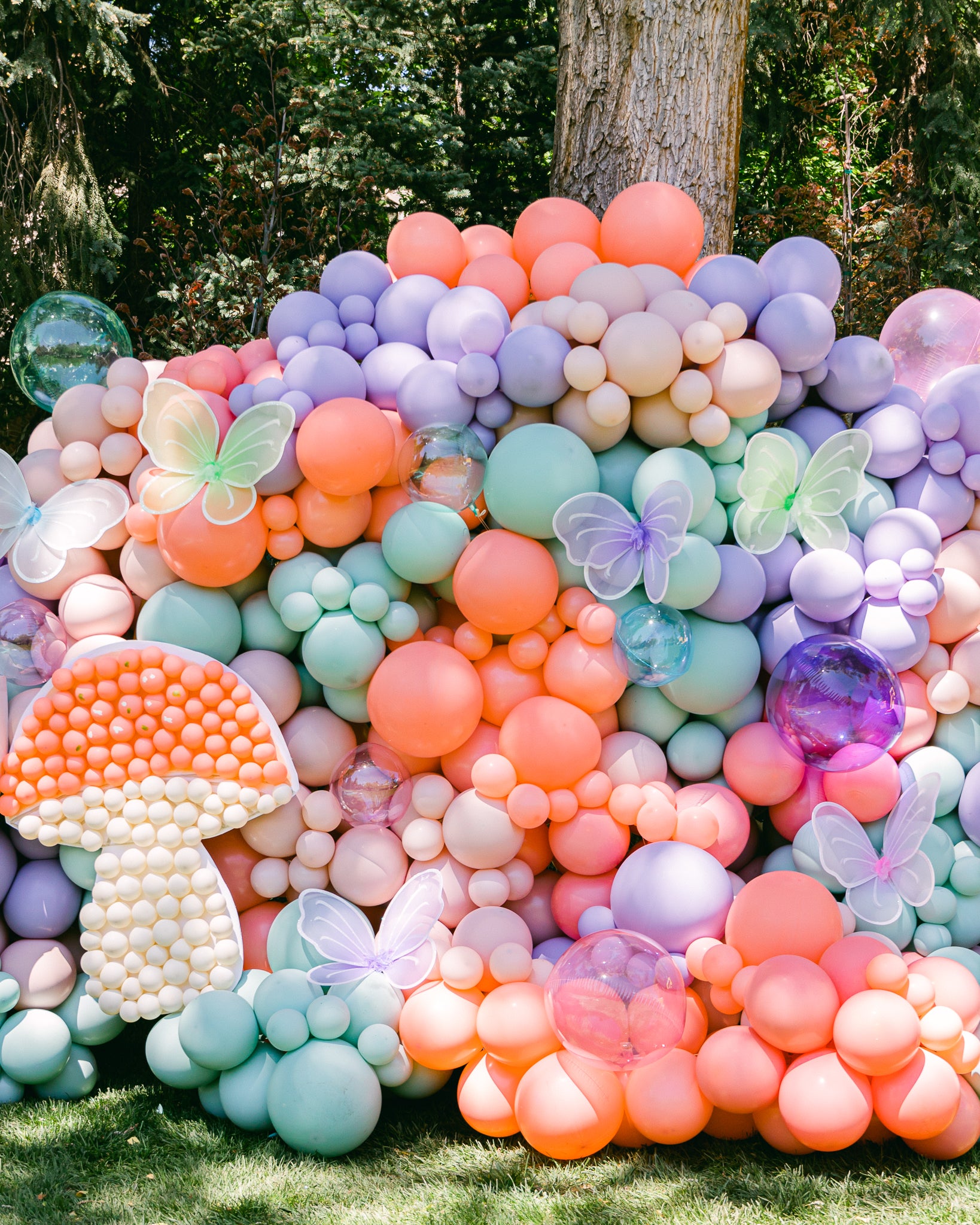The image showcases an elaborate outdoor scene featuring a striking balloon display set against a tree trunk with dense green foliage in the background. This vibrant display consists of a multitude of pastel-colored balloons of varying sizes, including orange, green, purple, and pink hues, as well as creamy beige and translucent spheres that resemble bubbles. The balloons range from large to tiny, creating a dynamic texture across the scene. Intermixed with the balloons are delicate fabric and wire butterflies, adding an ethereal touch.

A prominent feature in the arrangement is a mushroom-shaped structure made entirely of small balloons, with a red cap and white stem, positioned towards the left side of the display. Various clear, reflective balloons contribute to the whimsical aesthetic, giving a bubble-like appearance. The scene is further adorned with star-like dots on some of the translucent balloons, enhancing the magical forest ambiance complete with green leaves and grass at the base. This intricate setup suggests a carefully crafted photo backdrop or art installation intended to evoke the charm and wonder of a fairytale setting.